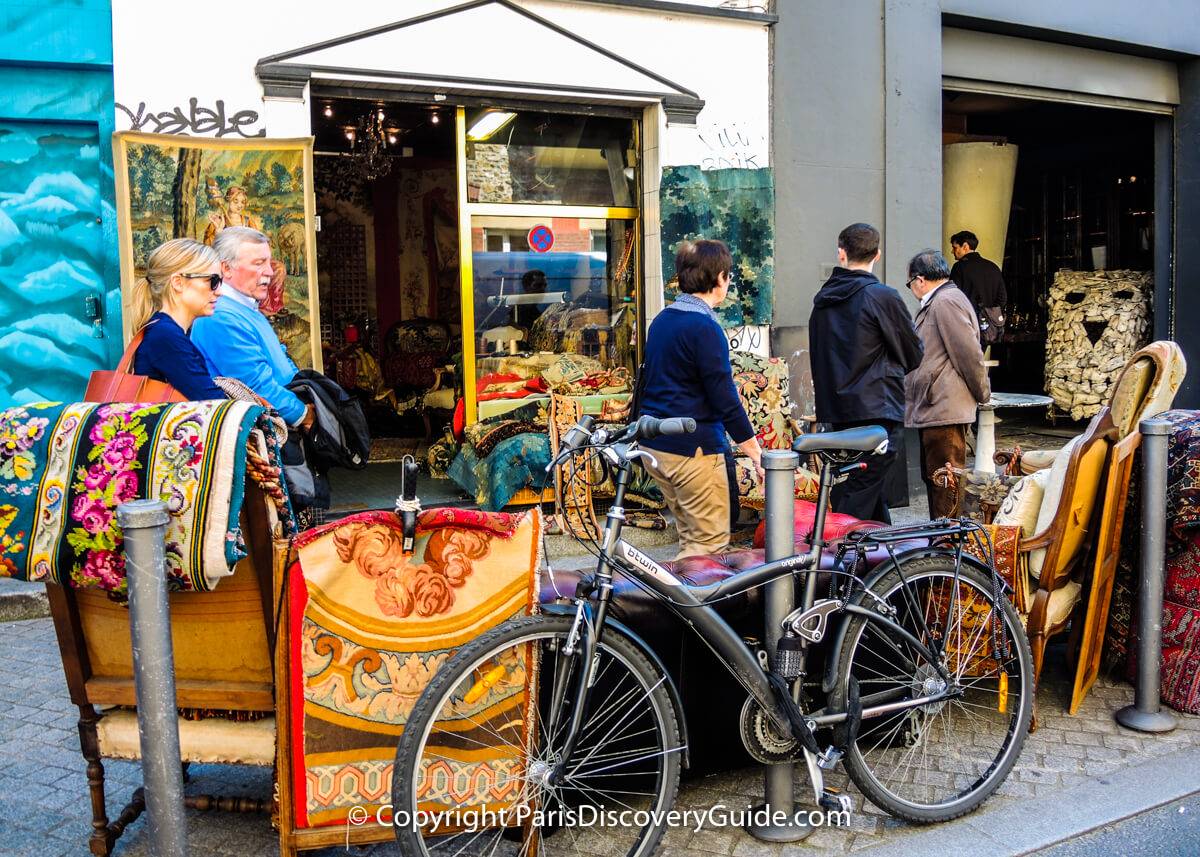The image features a bustling street scene outside a rug shop, with a variety of vividly colored rugs prominently displayed to attract customers. Several people, including what appears to be an older man and his daughter, a young man by himself, and a young man with his father, are examining the merchandise. The shop is adorned with an eye-catching mix of colors, including bright orange, red, purple, green, and various shades of blue. One rug stands out with its orange-red hue, while another is more intricate with purple flowers and green leaves against a dark blue background.

In the foreground of the image, there is a bicycle leaning against a dark brown leather sofa, suggesting a casual and lively atmosphere. The backdrop of the market is accented by a mixture of light blue designs and graffiti on the building walls. The scene is filled with a spectrum of colors, including gray, black, white, pink, pewter, and silver. The bottom center of the image bears the text, "© parisdiscoveryguide.com," marking the photograph's copyright and origin.